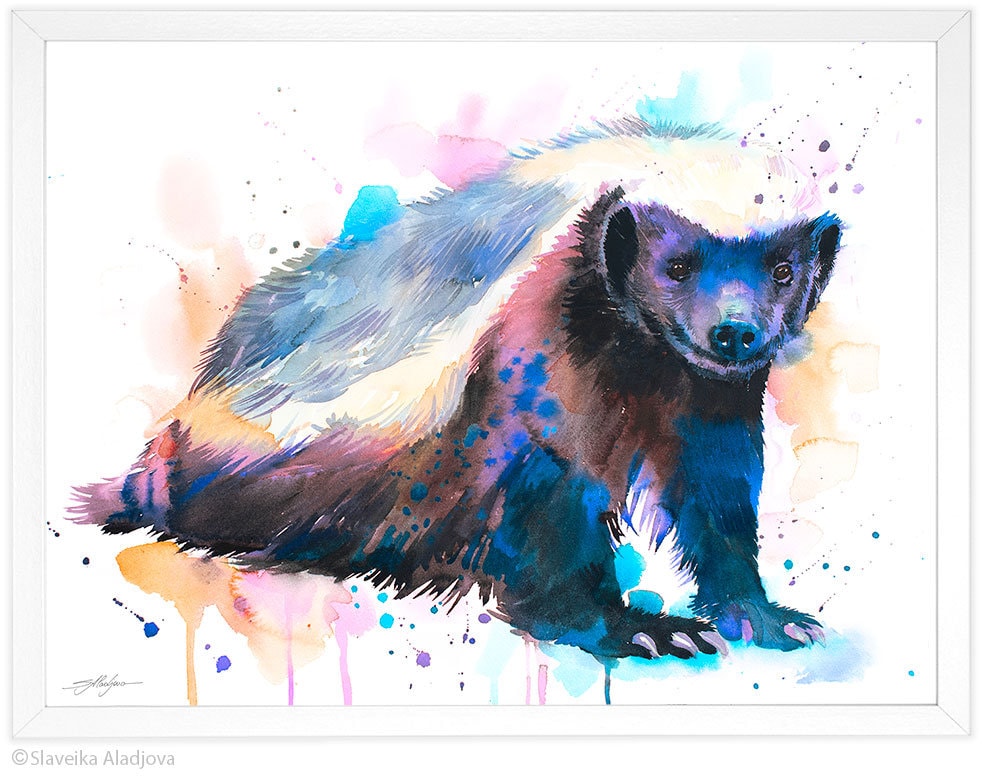This horizontal rectangular watercolor painting features a vividly multi-colored bear, which some may mistake for a badger due to its distinctive coloring and style. The bear is depicted in a seated position with its back legs sprawled out, while its front legs are propped up as though performing a push-up. The bear’s front legs are painted blue, while the visible shoulder is an orange hue. The face is rendered in dark tones, contrasted strikingly with what resembles a cape draping over its head and down its back. This "cape" transitions from white around the edges to patches of pink, yellow, and blue on its back. The bear’s overall body incorporates various shades including purple, red, turquoise, and green, giving it a surreal and dynamic appearance. It is positioned to the right of the image, with its head turned to face the viewer, and appears predominantly white on top and black below. Surrounding the bear are smudges and drips of paint, adding to the abstract aesthetic. The piece features the artist's signature, located in the lower left corner, identified as "Copyright Slaweka Aladjovea." The artwork is framed by a white border, enhancing its vibrant and artistic impact.